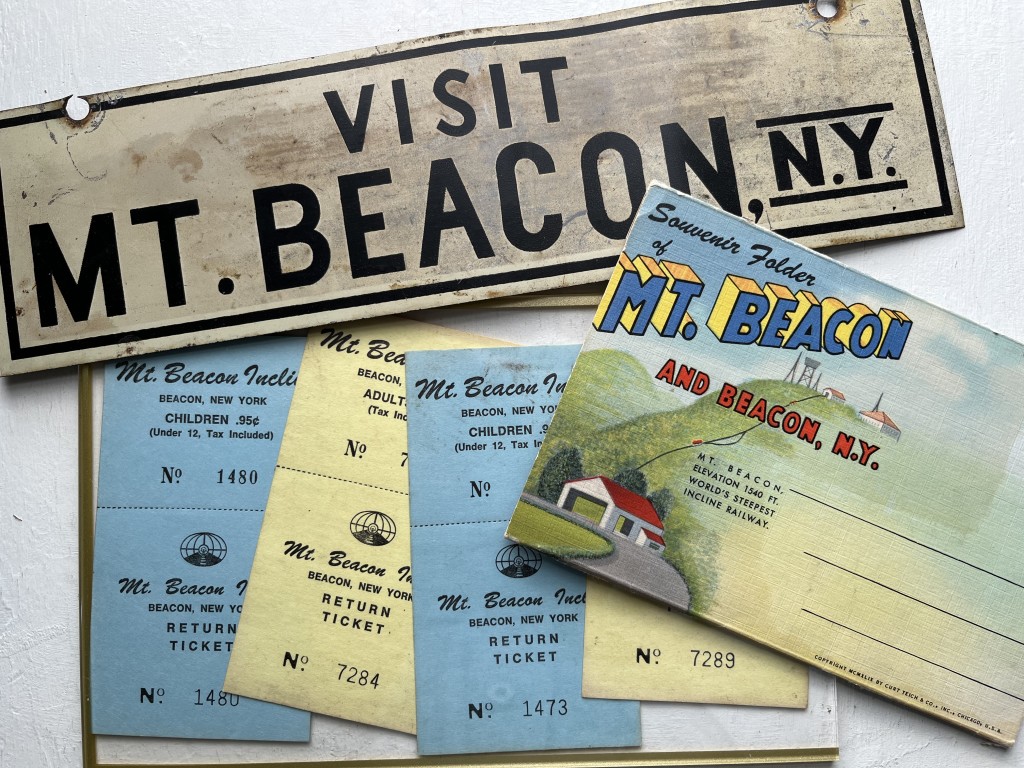The photograph depicts a vintage advertisement for Mount Beacon, New York. At the top center, there's an aged, slightly angled metal sign that reads, "Visit Mount Beacon, NY" in prominent black letters. Beneath this sign, a nostalgic mailer overlays it, labeled "Souvenir Folder of Mount Beacon and Beacon, NY," embellished with decorative blue text. This mailer showcases an image of two red-roofed buildings situated on a hillside, accompanied by metallic structures resembling a water tower. A long wire descends from these buildings, connecting to another structure with a red roof at the hill's base. Further below, four alternating blue and yellow tickets for the Mount Beacon Incline are displayed, each marked with unique numbers. The blue tickets are identified as children's return tickets priced at 95 cents, including tax, while the yellow tickets are presumably for adults. The overall arrangement conveys a nostalgic collection of postcards, signs, and tickets, capturing the essence of exploring Mount Beacon.